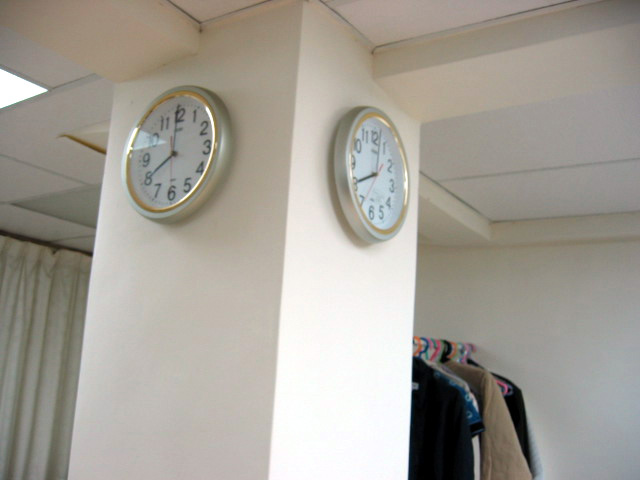In the image, we see a photograph taken inside a white room, possibly a personal space or a department store. Centrally positioned in the room is a square pillar extending from the ceiling to the floor. The point where the pillar's corner faces the camera is clearly visible. On the left side of the pillar, white drapery hangs down, while on the right, a silver metal bar extends from the other side of the pillar to the wall, supporting various pieces of clothing on hangers. The hangers are of multiple colors including white, blue, dark blue, and pink, suggesting a personal collection rather than a professional retail display.

Notably, there are identical round clocks on each visible face of the pillar. Each clock features a gold frame around the outer edge, a white clock face, black numbering from 1 to 12, and black minute, hour, and second hands. Both clocks display the time of 8:00; one clock's second hand points to 35 seconds, and the other to 29 seconds. Additionally, a fluorescent recessed light is partially visible at the top left corner of the photo, contributing to the bright illumination of the room. A clothing rack is positioned in the bottom right-hand corner, holding garments in blacks, tans, and blue hues.